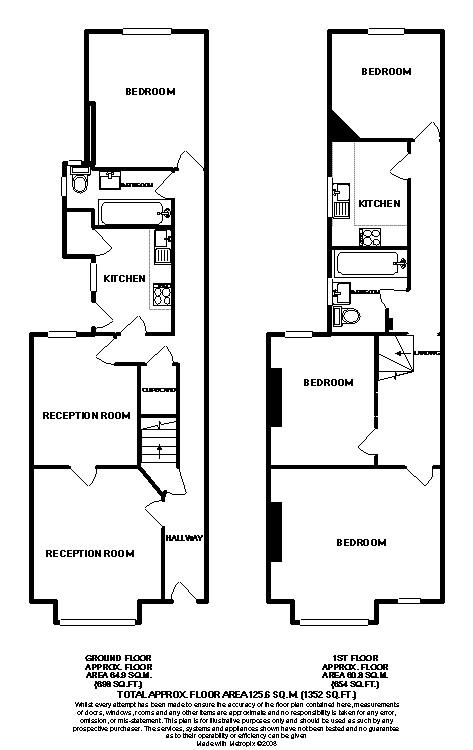Black and White Floor Plan of a Two-Story Building

This detailed, black and white floor plan illustrates a two-story building consisting of a ground floor and a first floor. The ground floor has an approximate floor area of 649 square meters (approximately 698 square feet), while the first floor covers an approximate area of over 600 square meters. The total floor area for both levels is 125.6 square meters (1,352 square feet).

The ground floor features a lengthy hallway that connects various rooms, including two reception rooms, a kitchen, and a bedroom. There are closet spaces situated along the hallway for storage purposes.

The first floor primarily houses multiple bedrooms and additional functional spaces. There are at least two bedrooms, aligned similarly to the reception rooms below. There is a staircase leading from one of the bedrooms to the first floor, adjacent to a bathroom. Another kitchen is surprisingly located on this floor, which might suggest the building could potentially accommodate two separate living areas or units.

Overall, the floor plan offers a rather simple yet functional layout suitable for versatile living arrangements.